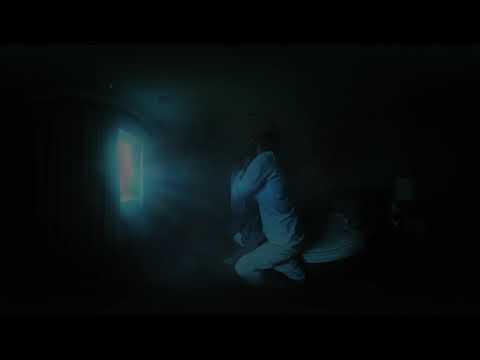In a photograph that appears dark and somewhat grainy, there is a person clad in a long sleeve white shirt and white or khaki pants, positioned centrally against a predominantly black background. The image captures them in a peculiar, dynamic stance, with one knee bent forward and the other leg extended back, almost as if in mid-lunge. Their black hair frames an obscured face, adding to the mysterious ambiance. 

To the left side of the image, a vivid turquoise blue light emanates from a square window, casting an ethereal glow across the room and onto the person, further illuminating their outline. The bright rays from this window faintly trace patterns on the ceiling and adjacent walls, contrasting the surrounding darkness.

In the background, a white bed can be discerned, although its details are somewhat faint. Nearby, there seems to be an object resembling a white table lamp. The overall image is encased in a circular frame of black, intensifying the focus on the brightly lit center where the person, mesmerized by the light from the window, stands against the backdrop of an otherwise pitch-black room.